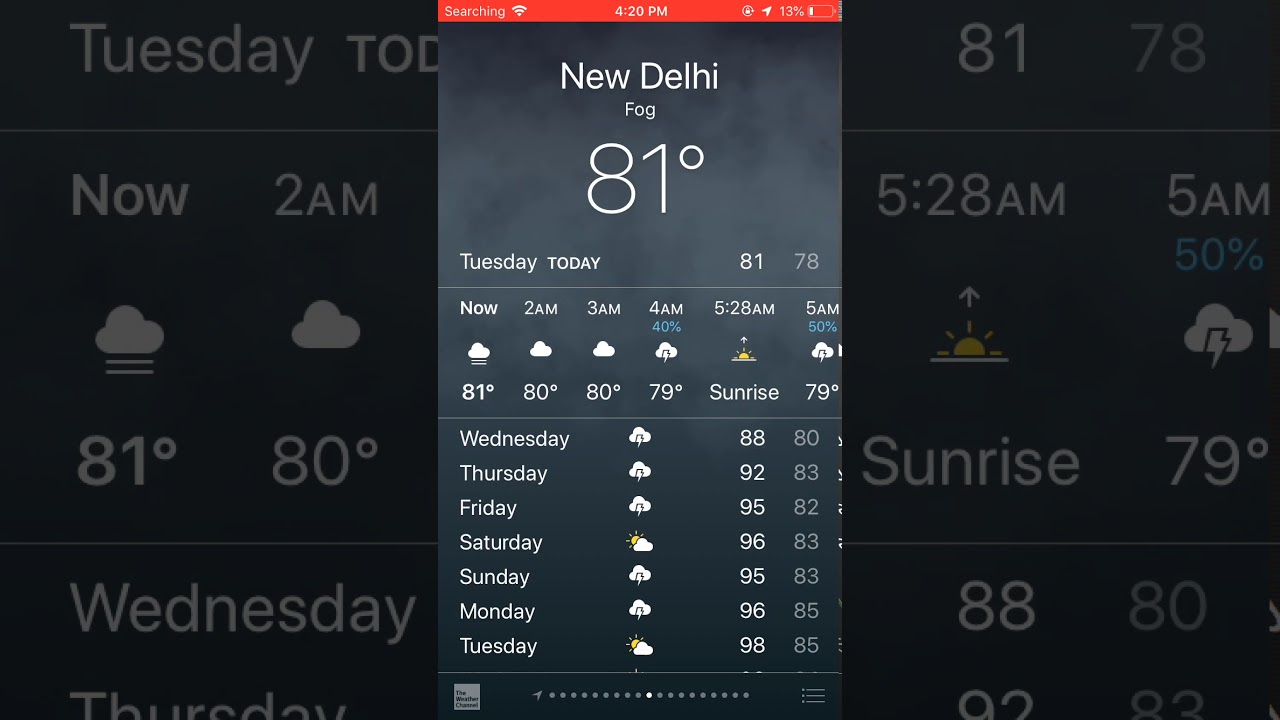This is a detailed screenshot of a weather app displayed on a cell phone, evident from the battery bar, signal search icon, and the current time visible at the top. The top bar of the screen is strikingly red with bold white font that immediately catches the eye. Below this, on a gray, chalkboard-like background, the name of the city, New Delhi, is displayed prominently in white font, indicating the location. 

Directly underneath the city name, the current weather condition is marked as "fog" in white font, reflecting the atmospheric status in New Delhi, India at the time the screenshot was taken. A large "81°" symbol is showcased below, providing a clear and immediate reference to the current temperature in New Delhi.

Further down, the app displays the day, "Tuesday," along with a detailed hourly forecast for the entire day. This section allows users to view specific weather conditions, chances of rain, and sunrise times at various hours, enhancing the app's utility for planning purposes. At the very bottom, the app includes an extended forecast, offering a preview of the weather for the upcoming days, thus facilitating long-term planning.